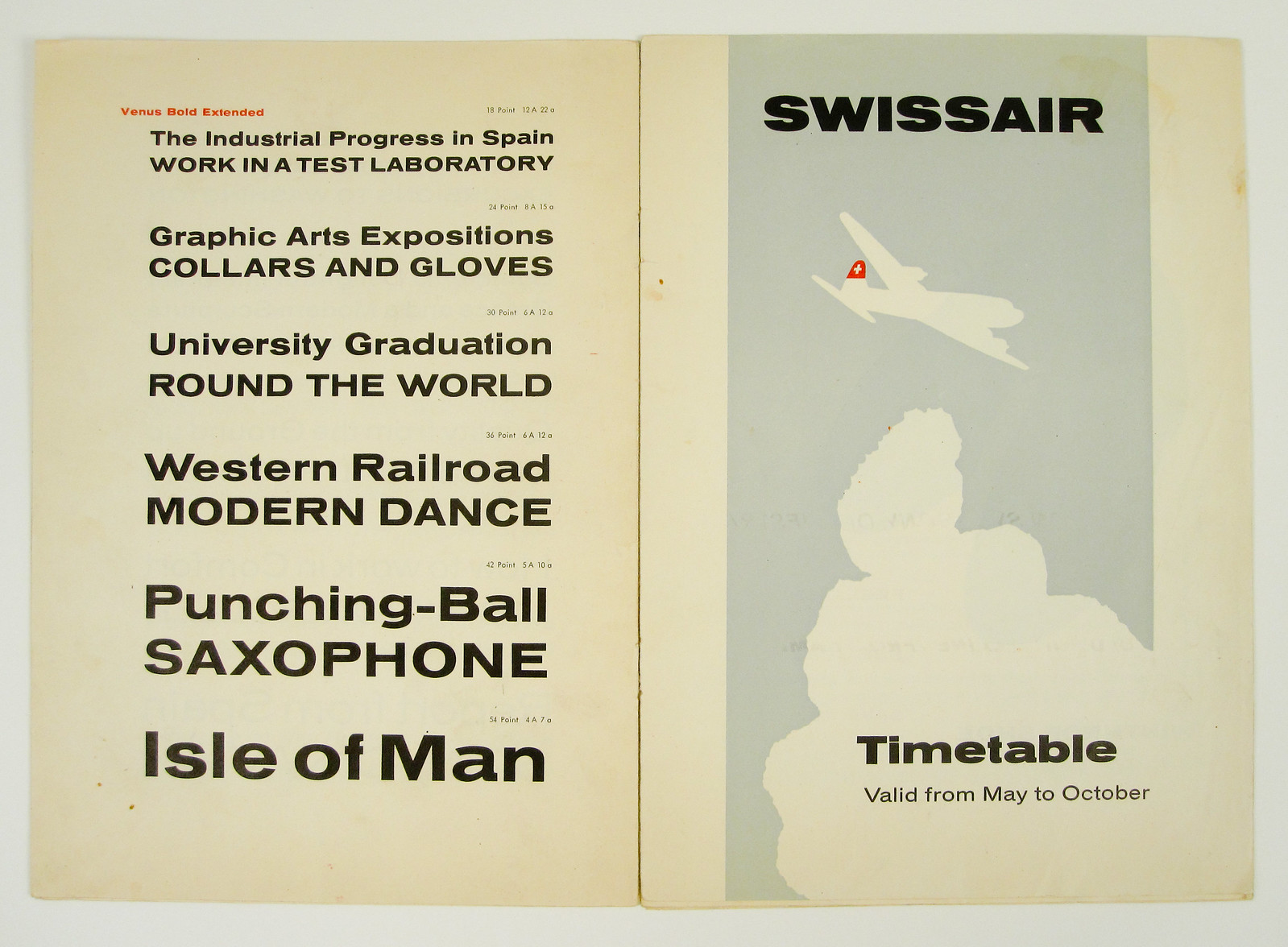This color photograph showcases a horizontal landscape-oriented, vintage print production piece, presented as an open two-page spread resembling an old handbill aged to a beige hue. The left side of the spread features various article headlines in black text, descending in size from top to bottom. Headings include "The Industrial Process of Spain," "Work and Test Laboratory," "Graphic Arts," "Collars and Gloves," "University Graduation Around the World," "Western Railroad," "Modern Dance," "Punching Ball," "Saxophone," and "Isle of Man." The right side contains an illustration of a white airplane with a red Swiss Air logo on its tail, soaring in a blue sky dotted with white clouds. Above the plane is the bold black text "Swiss Air," and in the bottom right corner are the words "Timetable valid from May to October." The print appears to be a digitally created or printed piece with spot color, contributing to its aged, vintage aesthetic.